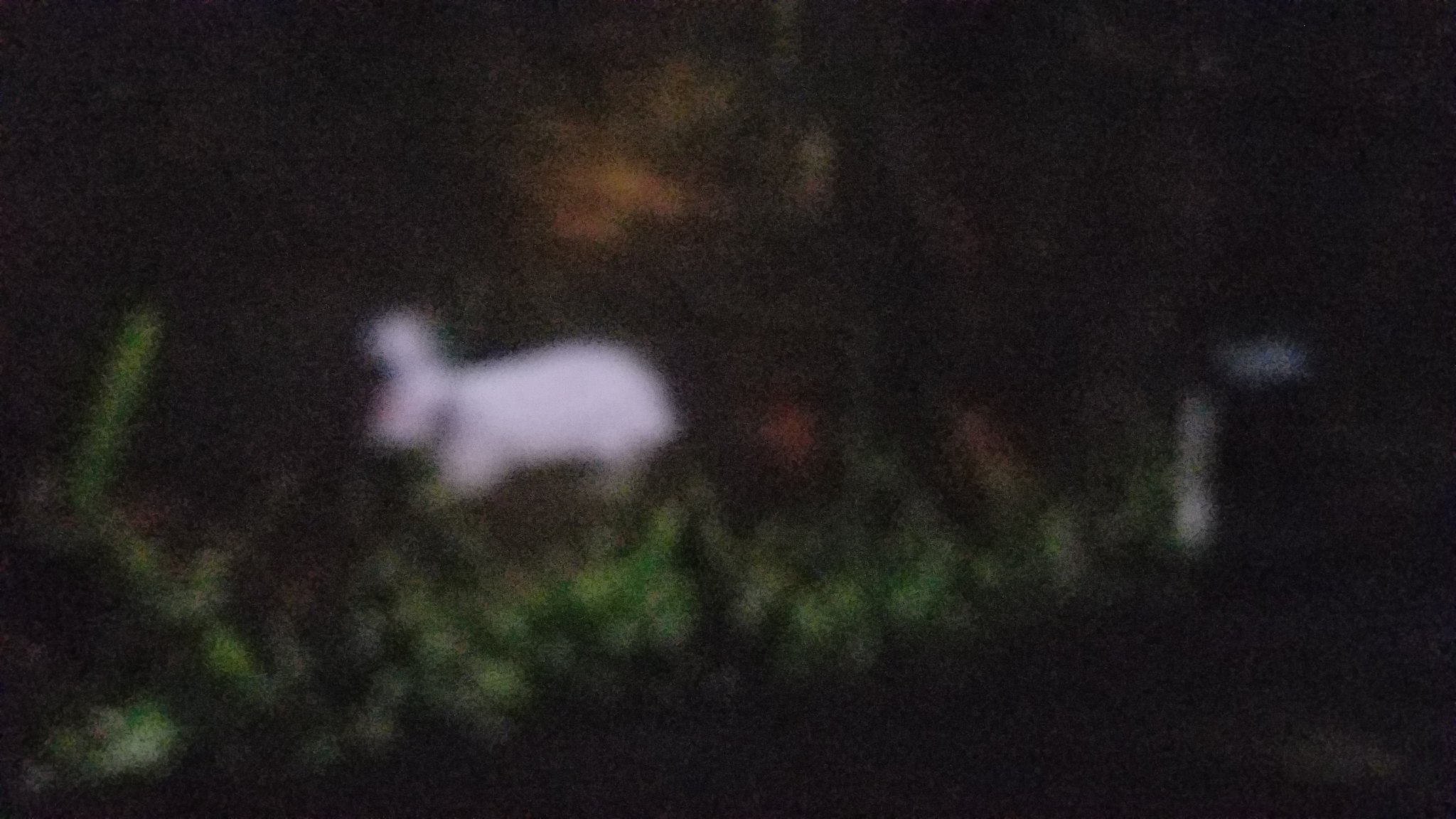A grainy, blurry photograph captures an indistinct scene of a garden or forest at dawn or dusk, with an overcast light suggesting the time might be either sunrise or sunset. In the midst of this natural setting, amidst patches of grass, tall leaves, and bushes, a small white creature—possibly a rabbit or a dog—stands out. This creature appears to be wearing a dark collar around its neck. In the background, a faint, dirt path winds through the vegetation, adding depth to the otherwise obscure image.